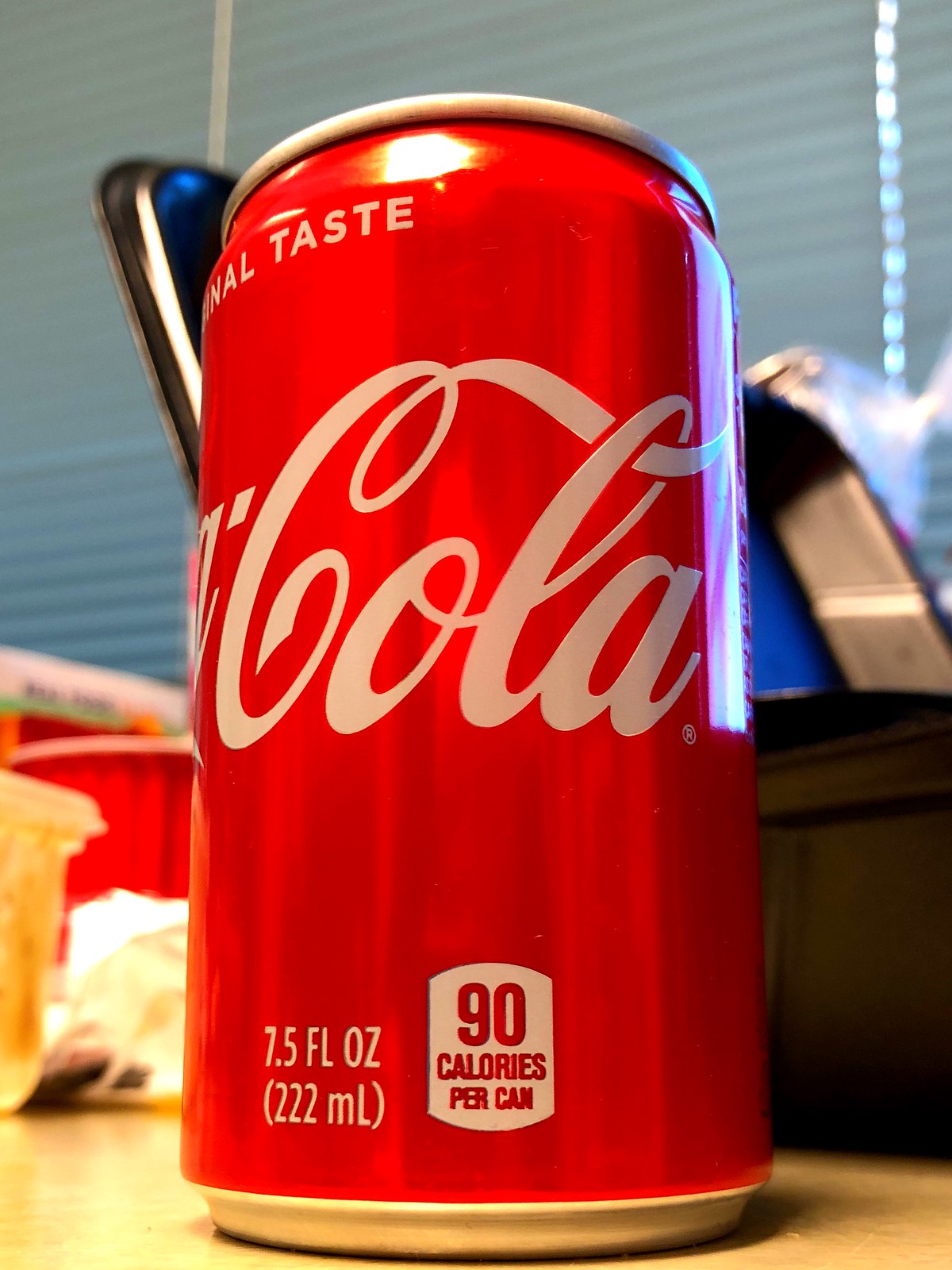This image features a classic red Coca-Cola can prominently displayed on a beige countertop. The iconic Coca-Cola logo is showcased in white script across the middle of the can, which holds 7.5 fluid ounces (222 mL) of the beverage. A label at the bottom of the can indicates it contains 90 calories. Encircling the top of the can, "Original Taste" is written in bold white capital letters. The background reveals a dark brown wooden shelf or counter, adding a rustic touch to the scene. Nearby on the countertop are additional items: notably, a Tupperware bowl containing a yellow substance and a red cup positioned slightly behind the Coca-Cola can, contributing to the everyday atmosphere of the setting.